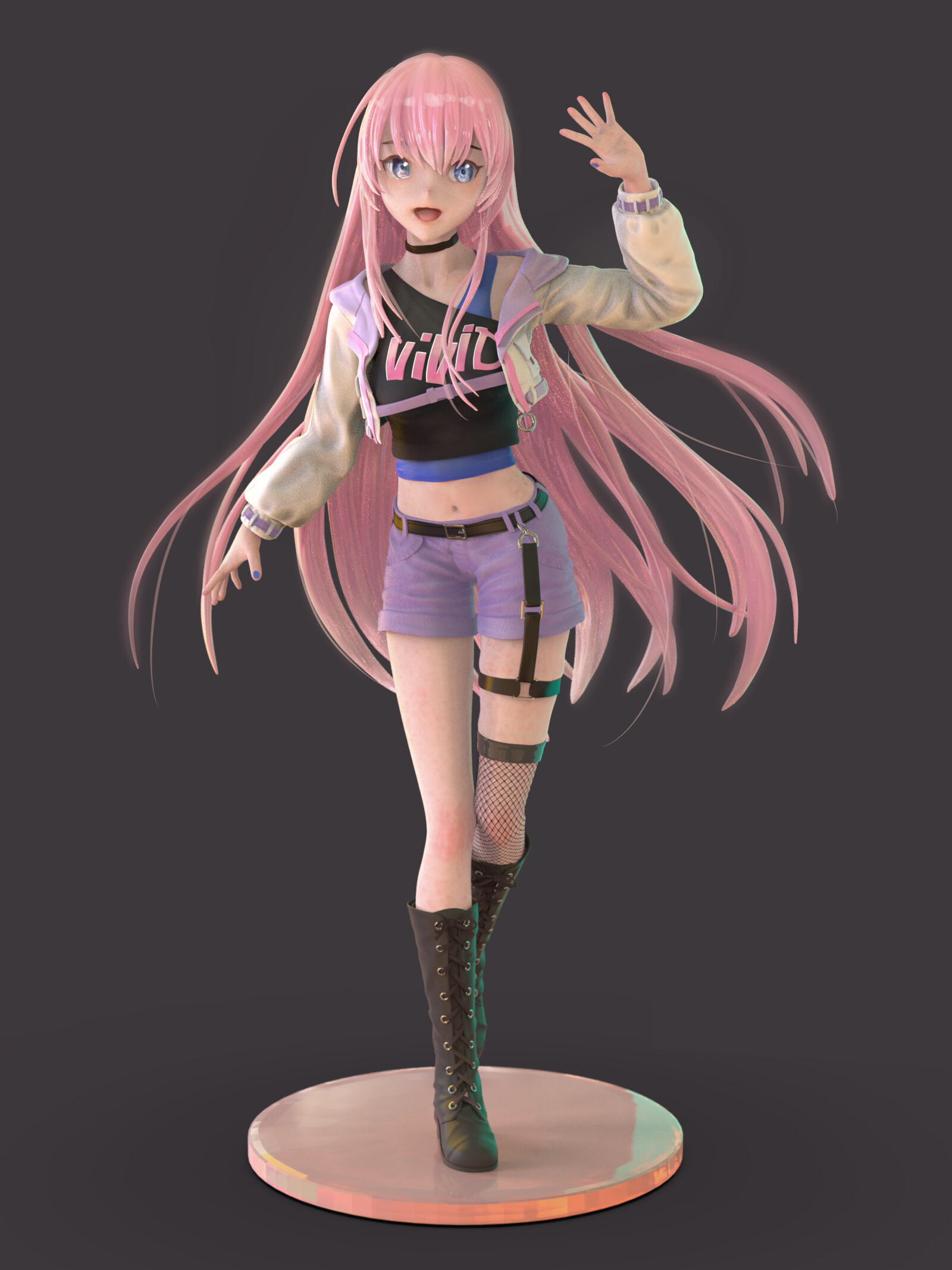This is a highly detailed, computer-generated illustration of an anime-style female character standing on a pink pedestal within a black background. She sports long, flowing pink hair with long pink bangs and big crystal blue anime eyes. Her outfit consists of a black choker, a short white jacket with pink and purple highlights on the lapel and sleeves, layered over two tank tops: a black one with the word "Vivid" emblazoned in pink across the chest, and a periwinkle blue one beneath it. Her midriff is exposed, revealing a strap from her belt loop extending down to a garter-like area on her thigh. She is dressed in short, cuffed purple shorts with a black belt, and on her left leg, she wears a partial fishnet stocking. Her footwear includes high, black, laced-up boots that reach her knees. Additionally, her nails are painted with pink and purple polish—pink on most fingers and purple on both thumbs. The composition gives the impression of movement, with her hair flowing backwards as she stands in a striking pose.